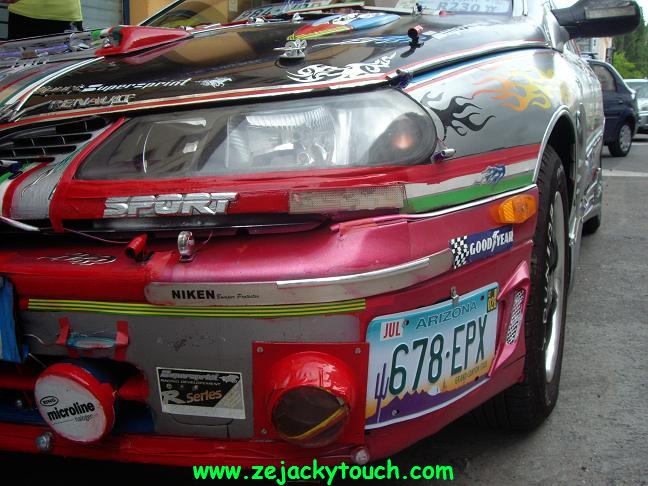This close-up image features the driver's side headlight of a modified Renault racing vehicle. Dominating the scene is the Arizona license plate, numbered 678EPX with an expiration date in July, prominently mounted along the red bumper. The car itself is primarily silver, with a contrasting black hood and vivid, visually striking little flame decals extending from the headlight and wheel well. The sporty aesthetic is further emphasized by a "SPORT" tag situated below the headlight. The bumper and vehicle surface are festooned with a significant number of stickers, including distinguishable ones from Goodyear, Niken, Microlign, and www.zjackytouch.com, making it clear that the car is heavily sponsored. In addition, the tires are solid black. The outdoor setting is a paved concrete road surrounded by other vehicles in the background, adding context to the scene. An interesting detail is that there are two additional license plates placed on the dashboard, barely visible at the top of the frame. The car's varied color palette includes red, black, silver, and smaller accents of blue, green, pink, purple, orange, yellow, white, and gray, which contribute to its vibrant and eye-catching appearance. Some minor damage can also be observed on the car’s surface.